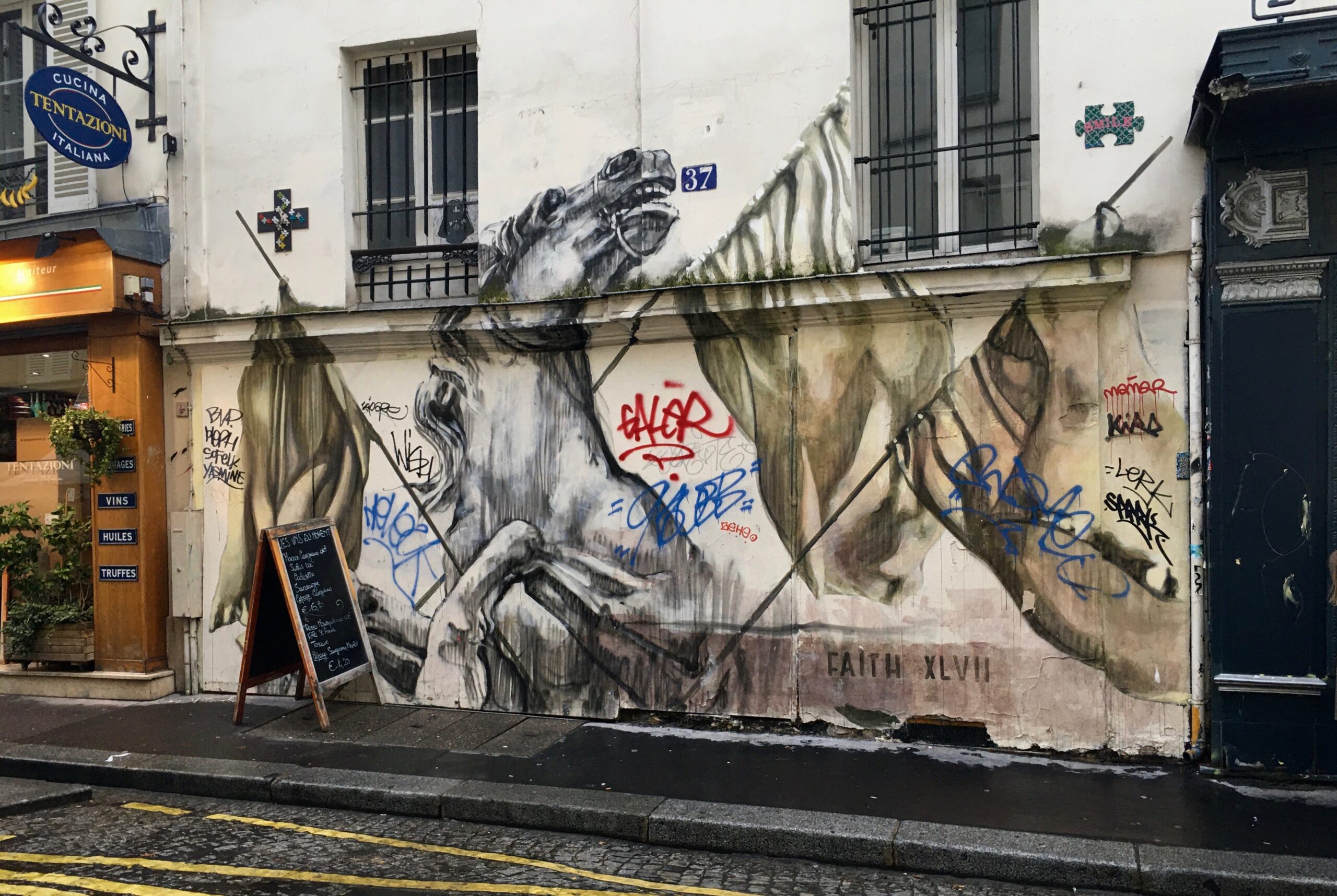This color photograph captures a vibrant mural painted on the white wall of a building located on a cobblestone street with an asphalt sidewalk. The focal point of the mural is a dynamic image of a horse with its front legs raised, its head thrown back, and its mouth open as it gazes towards the upper right. Surrounding the horse are several white flags with black poles. The building features two windows, each secured with black bars, and a blue plaque with the number 37 in white letters. On the right-hand side of the image, there is a black door, and to the left of the building is a restaurant with a blue sign reading "Cucina Italiano Tentaziano" in white and yellow lettering. A small chalkboard sign stands in front of the restaurant. Additional details in the mural include a hand holding the flags, a cross, and a few puzzle pieces, enhancing the eclectic street art scene.